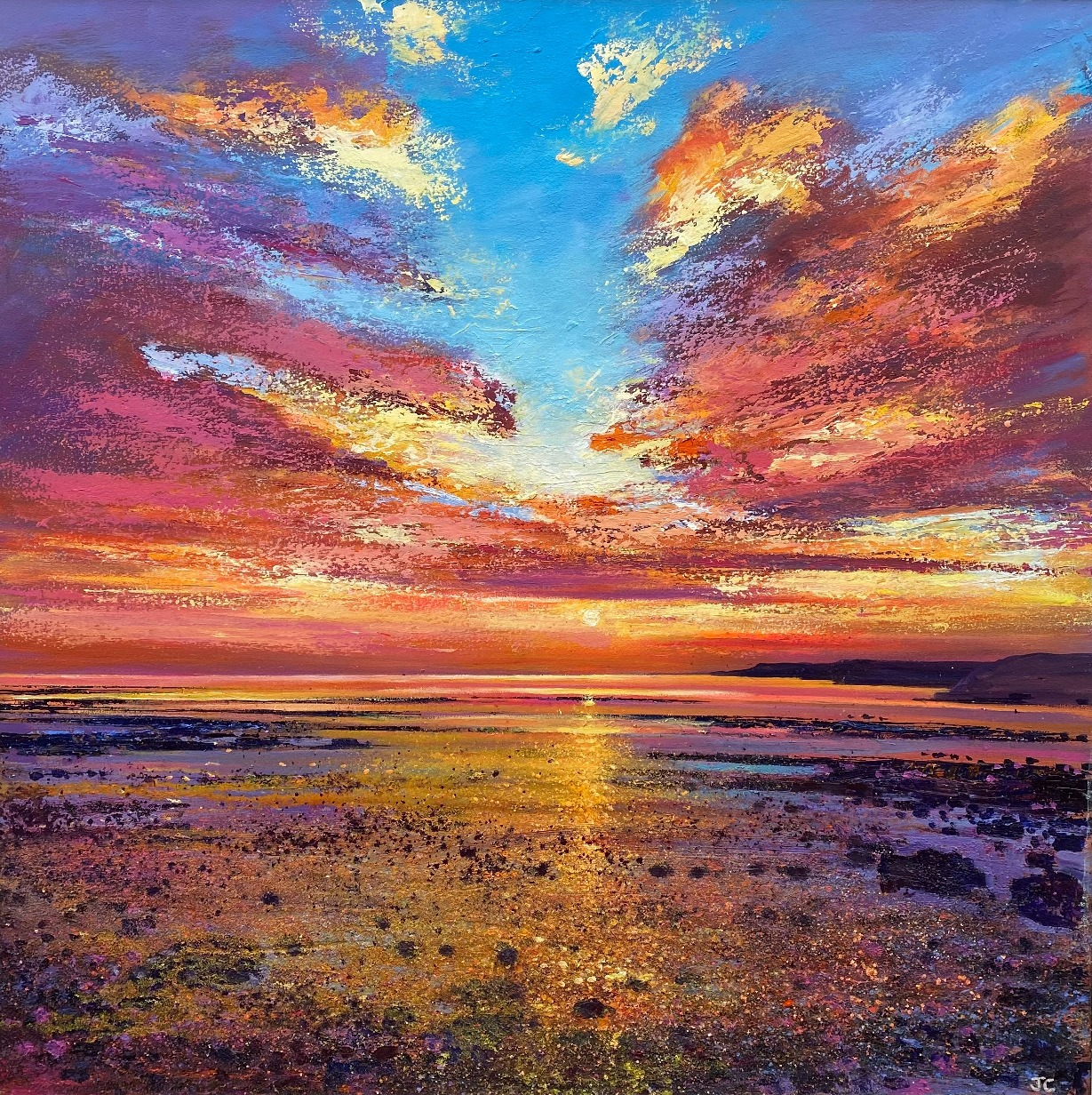This artwork depicts a stunning sunset with a dynamic array of colors and intricate details. At the top of the painting, a streak of light blue descends about halfway from the center, flanked by clouds that part to reveal more blue sky. Moving left to right, the sky transitions from light yellow and orange hues to deeper pinks and purples as it extends outward. 

The sun, represented as a bright yellow dot in the central part of the scene, casts a radiant line of light straight across the painting. This light further enhances the color transition in the sky, while also creating a striking reflection on the water below. The water itself mirrors the sky's coloration, ranging from bright yellows near the center to deeper pinks and purples as it moves outward. The gentle waves in the water display a variety of purple shades, contributing to the overall depth and texture of the scene.

At the base of the painting, the ground is depicted with dark, black rocks that add contrast to the vivid colors above. The central area, where the sun’s reflection hits, is notably brighter, with yellow tones that gradually darken as they spread toward the edges, meeting the black rocks and purple shades on the ground.

In the bottom right corner, the artist's signature, "JC," can be seen, subtly integrated into the composition. This meticulous and vibrant depiction captures the serene yet dynamic essence of a sunset, blending natural elements with an expressive color palette.